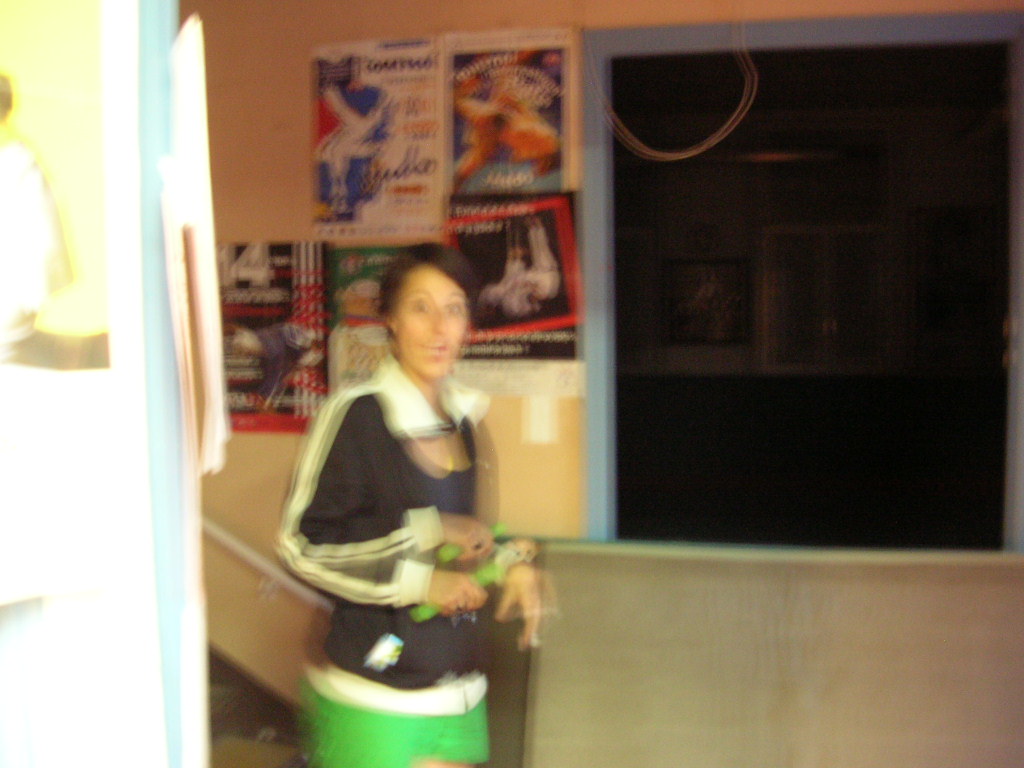This blurred image captures a moment of intense surprise on a woman's face as she descends a staircase. The background features a wall adorned with five posters—two on the top row and three across the bottom. A railing lines the wall, and below, a half wall reveals a dark, unlit room beyond. The woman, with short brown hair, is dressed in a green skirt or shorts paired with a black and white jacket that has a white collar and a low-cut top. Her eyebrows are raised, eyes wide open, and mouth agape, facing the camera clearly taken aback. Due to her movement, her arm appears blurred, giving the illusion of having two arms. She appears to be clutching some kind of doll or similar object adding an extra layer of curiosity to the scene.